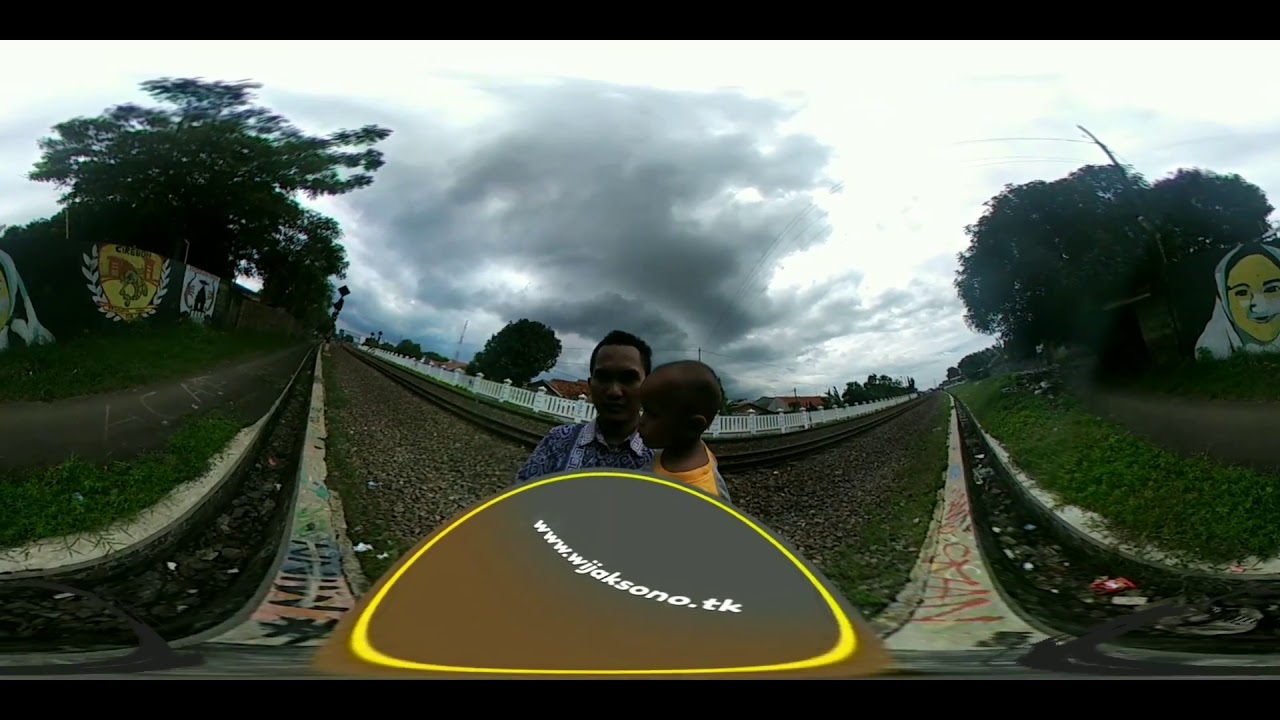In this outdoor photograph, a man with short dark hair, dressed in a purple paisley collared shirt, is holding a boy who is approximately four years old and dressed in a mustard-colored t-shirt. They are standing in front of a white picket fence with triangular caps. The image, seemingly taken using a fisheye or 360-degree lens, exhibits significant warping, especially around the trees on both the left and right sides. Behind them, there are railroad tracks that extend into the distance, featuring areas of light gray and darker cement. On the right side of the tracks, there is graffiti depicting a woman with a white shawl over her head, smiling at the viewer. On the left side, there are emblematic paintings, including a yellow one with fig leaves and another with a cat. Grass and sporadic trees populate the scene, and at the bottom of the image, partially obstructing the main subjects, a web address—www.wijaksono.tk—is visible in a circular, oval shape.